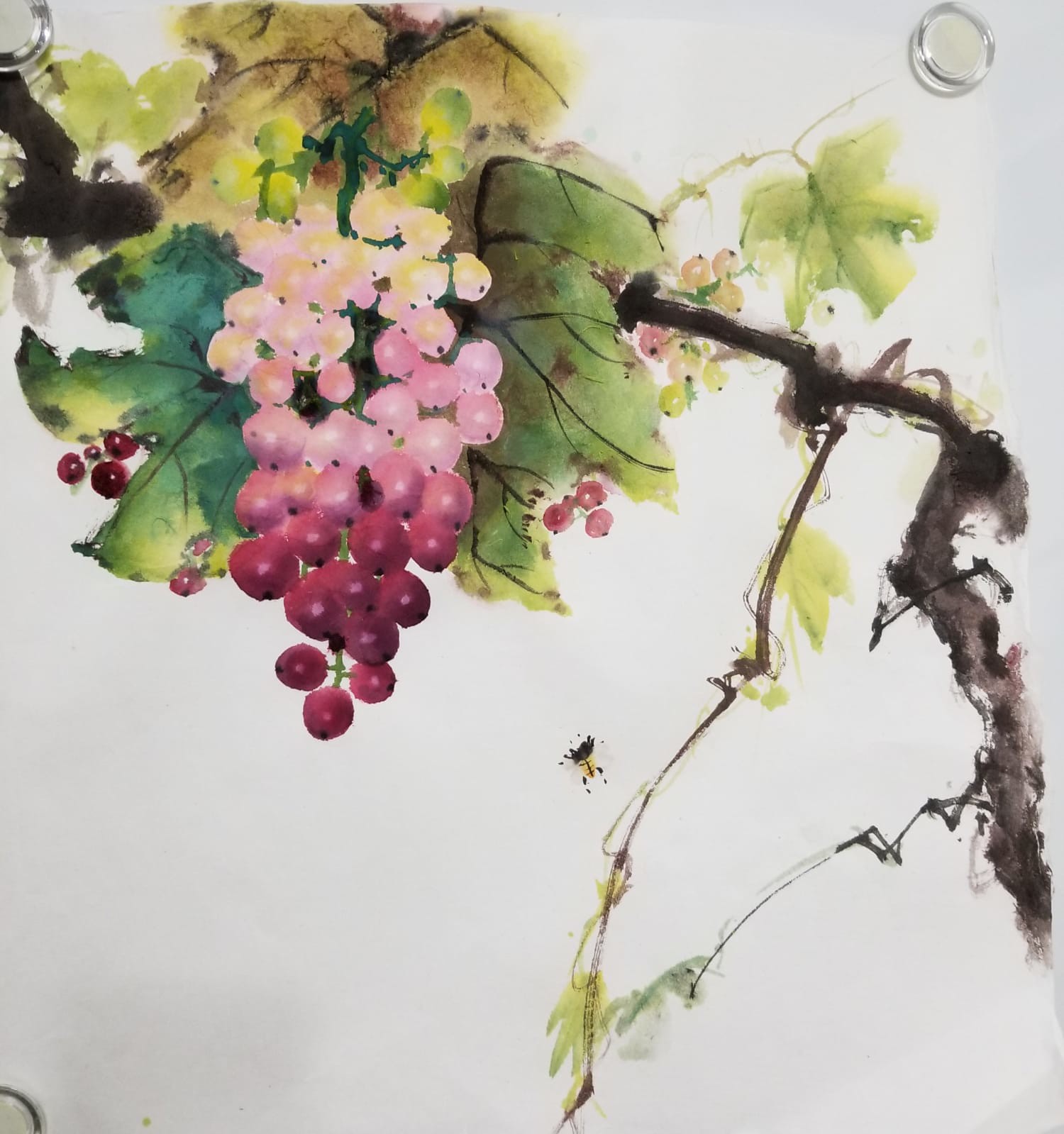The image depicts a detailed watercolor painting of a bunch of grapes hanging from a vine. Starting near the center-right, a thick brown branch extends upward, accompanied by a slightly thinner branch to its left. Both branches connect to clusters of light green and brown-green leaves. The grape bunch showcases a beautiful gradation of colors, with the upper grapes being a very light pink and yellow, the middle grapes a darker pink, and the ones at the bottom a purplish red, indicating varying levels of ripeness. In the upper right corner, a small silver circle is visible, adding a subtle metallic accent to the scene. Just below the grapes, to the right, there's a small detail resembling a tiny bee or bug, represented by a black speck with yellow underneath and minute black lines.